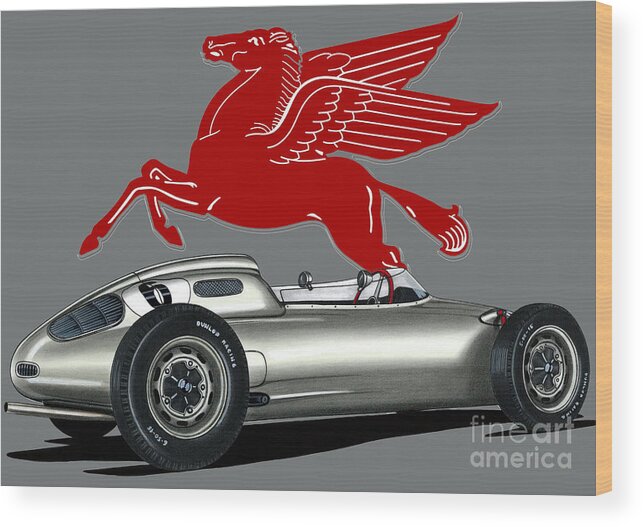This image is a highly detailed, stylized poster of a futuristic race car with a unique, silvery metallic finish. The car, a convertible with the top down, exhibits a sleek design with a curved, bubble-like rear end and is positioned such that the back is to the left and the front to the right of the image. It features large black tires, emblazoned with what appears to be "Dunlop Racing," and a prominent number six in a white circle on its trunk side. The steering wheel is strikingly red, and the car's headlights are situated right outside the seat area. The race car sits very low to the ground, enhancing its streamlined appearance.

Above the car, occupying nearly half of the upper part of the image, is a vivid red Pegasus—a winged horse—crafted with intricate, white etched details. The Pegasus seems to be either hovering or about to take flight, adding a sense of dynamic motion to the scene. The entire image appears to be printed on wood, with the side of the wooden block visible and painted tan, while the front showcases a medium-gray tone.

Overlaying the bottom right corner of the image is the branding "Fine Art America," signifying the art piece's origin. The combination of the race car's futuristic design and the mythological element of the Pegasus creates an arresting and imaginative visual.